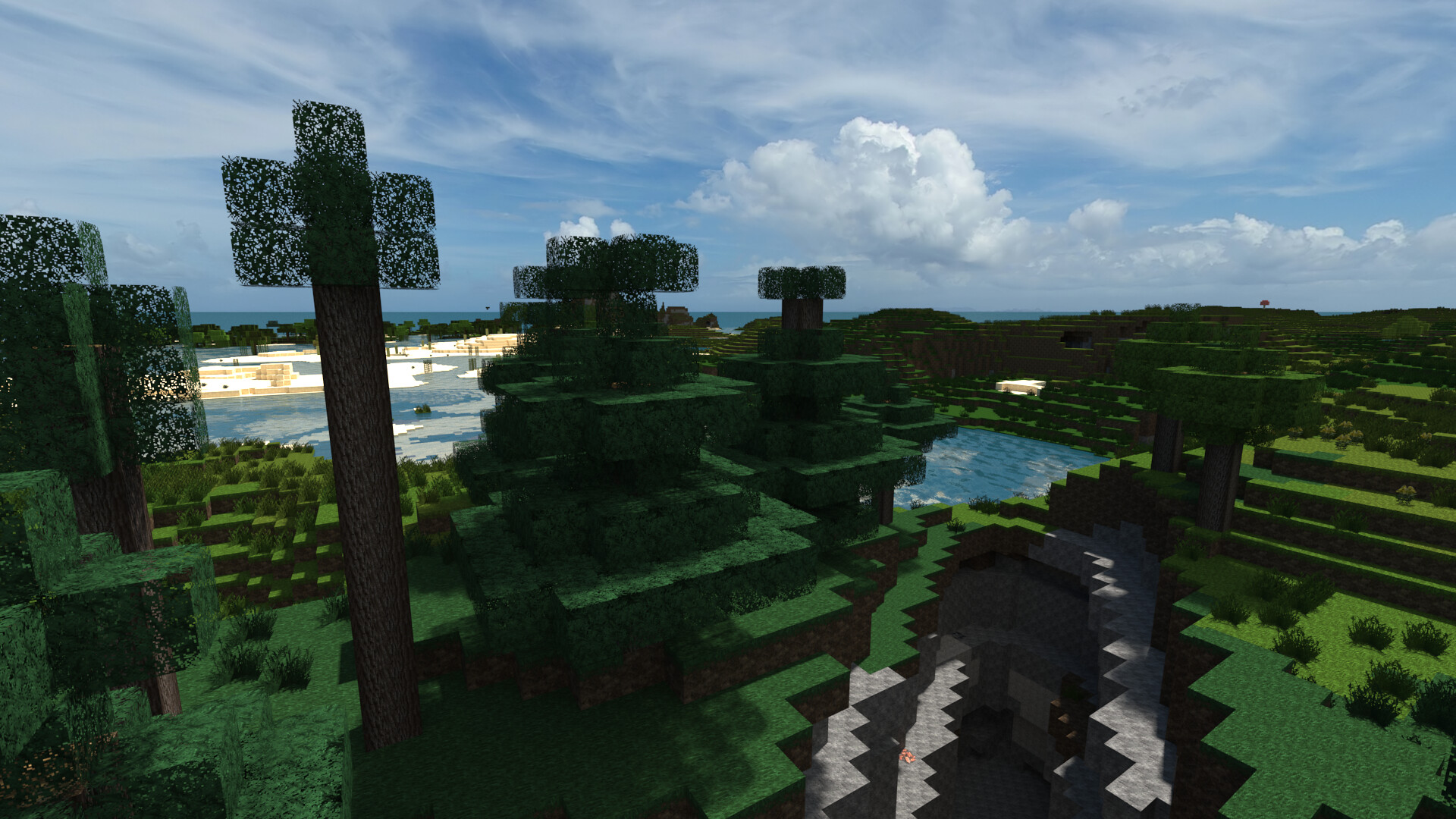The image is a screen grab from a pixelated video game, resembling Minecraft, featuring a vast landscape. The scene is composed of blocky, low-resolution textures depicting hills, grass, and plants. In the foreground, a large, humorously blocky tree stands to the left with a thick trunk and minimal leafy foliage represented by small, fuzzy blocks. On the right bottom side, there's a cave-like separation in the ground, featuring blocks that suggest concrete and a potential drop. The background showcases a tranquil ocean under a blue sky filled with clouds, lending a realistic, photographic quality to the scene. The lighting suggests it might be early morning or simply a cloudy day, capturing a serene and immersive outdoor environment.